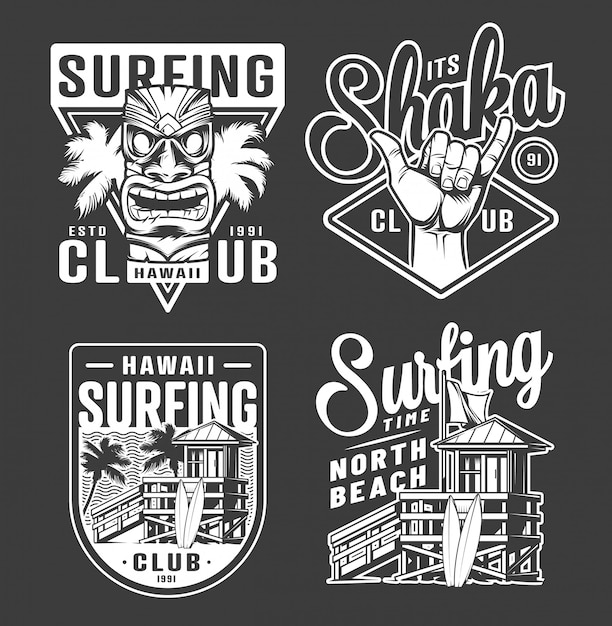This image features four distinct black and white graphics, prominently displayed against a dark gray background, resembling t-shirt designs commonly associated with a beach town aesthetic. The top left graphic reads "Surfing Club, Hawaii, established 1991," and features a tiki mask with palm trees extending from the sides. The top right graphic is labeled "It's Shaka Club" with a distinctive "91" circled on the right. The word "Shaka" is styled in dark gray cursive text with a white outline, accompanied by an illustration of a hand making the shaka sign, a familiar Hawaiian greeting. The bottom left graphic showcases a lifeguard stand with two surfboards leaning against it. Above, it reads "Hawaii Surfing Club, 1991." Finally, the bottom right graphic reads "Surfing Time, North Beach" in cursive text and depicts another lifeguard hut with a ramp on the left side, flanked by two surfboards and a flagpole with a white flag. Each design is centrally positioned and meticulously detailed, capturing various elements associated with surfing culture.